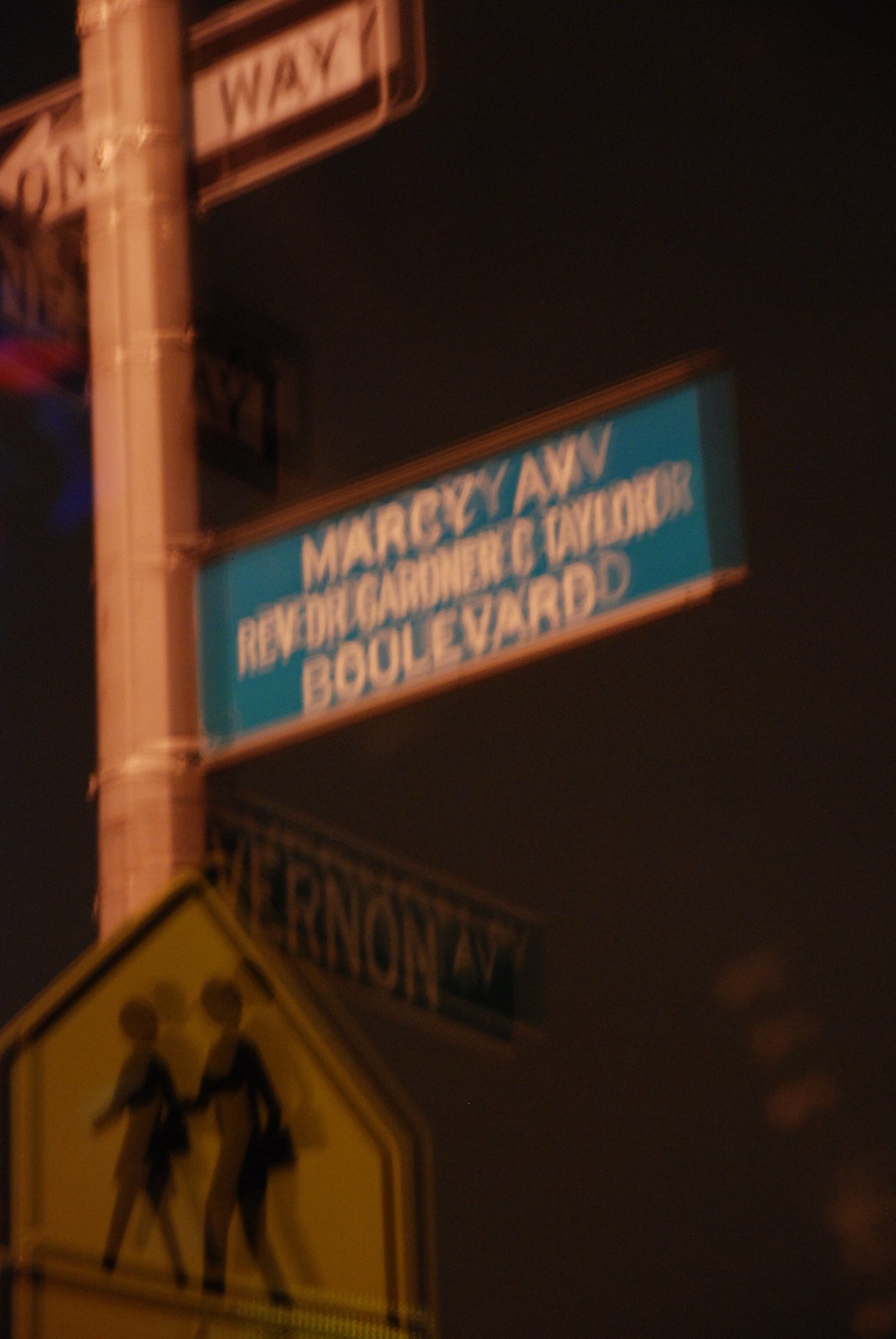The image captures a poorly taken, blurry nighttime photo of a street post crowded with multiple signs. At the top, a black-and-white "One Way" sign is barely legible due to the out-of-focus shot. Just below it, a light blue rectangular street sign displays "Marcy Avenue, Rev. Dr. Gardner C. Taylor Boulevard" in white text. Further down, a green street sign reads "Vernon Avenue." At the bottom, a yellow, five-sided pedestrian crosswalk sign features the silhouette of two people crossing. The dark, black sky is dotted with orbs, adding to the overall impression of an amateur photograph, with some of the text appearing doubled as if overlaid.